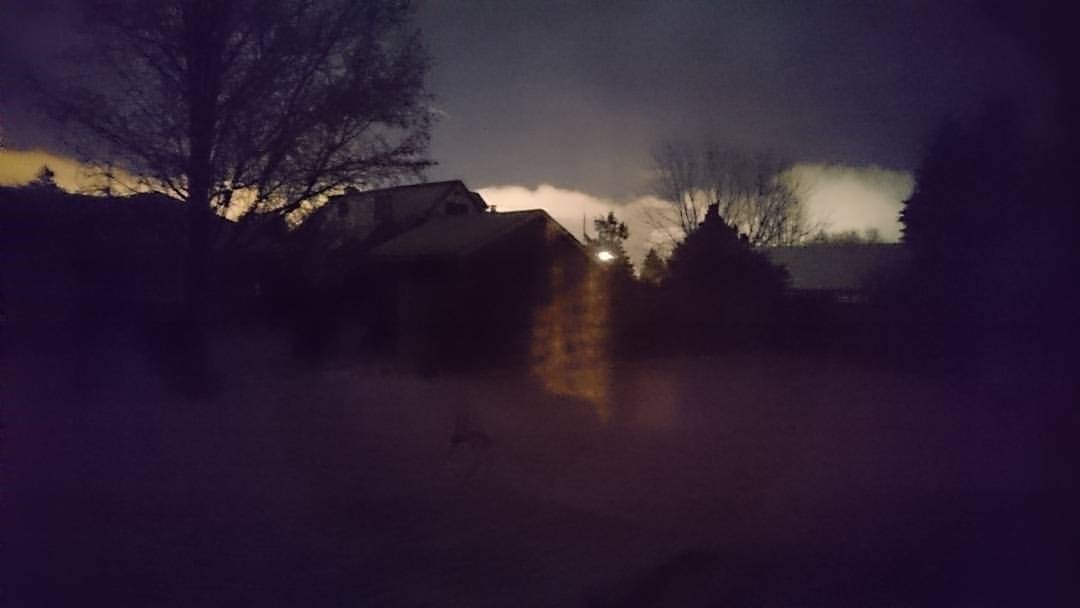This outdoor photograph, taken either at dawn or dusk, depicts a dark, somewhat gloomy scene with an old farmhouse-style home positioned just left of the center. The house features two peaked roofs and an illuminated lamp on the right side, casting a faint light pattern into the center of the image. The overall quality of the photo is grainy due to the low light.

The background is dominated by a dark gray, ominous sky with a line of white clouds cutting through the middle, adding a foreboding atmosphere. To the left of the house stands a tall tree, its shadow extending above the home and against the cloudy backdrop. On the right, there is a dense, bushy tree, and beside it, a tree that appears to have shed most of its leaves, almost blending into the dark backdrop.

Barely visible, a line of mountain tops peeks out with treetops above them, adding depth to the background. The lower half of the image is shrouded in a shadowy, almost mist-like foreground, contributing to the nebulous and mysterious ambiance of the entire scene.